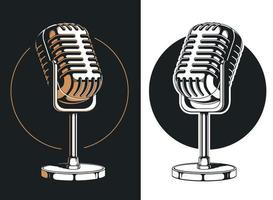This image features two side-by-side illustrations of vintage microphones set against contrasting backgrounds. Both microphones are mounted on silver stands with distinctive U-shaped tops and thick cylindrical bodies reminiscent of retro designs, featuring grill lines for sound diffusion.

The left illustration has a black background with a thin gold circular outline behind the microphone, which is slightly tilted towards the upper left corner. The microphone, displaying a monochromatic white color, is on a round base supported by a long rod.

In contrast, the right illustration presents a white background with a solid black circle behind the microphone. This microphone is also white but is tilted towards the upper right corner. The consistent position and design of the microphone across both images highlight the visual interplay between the contrasting black and white themes, emphasizing the microphone's classic aesthetic and functional architecture.